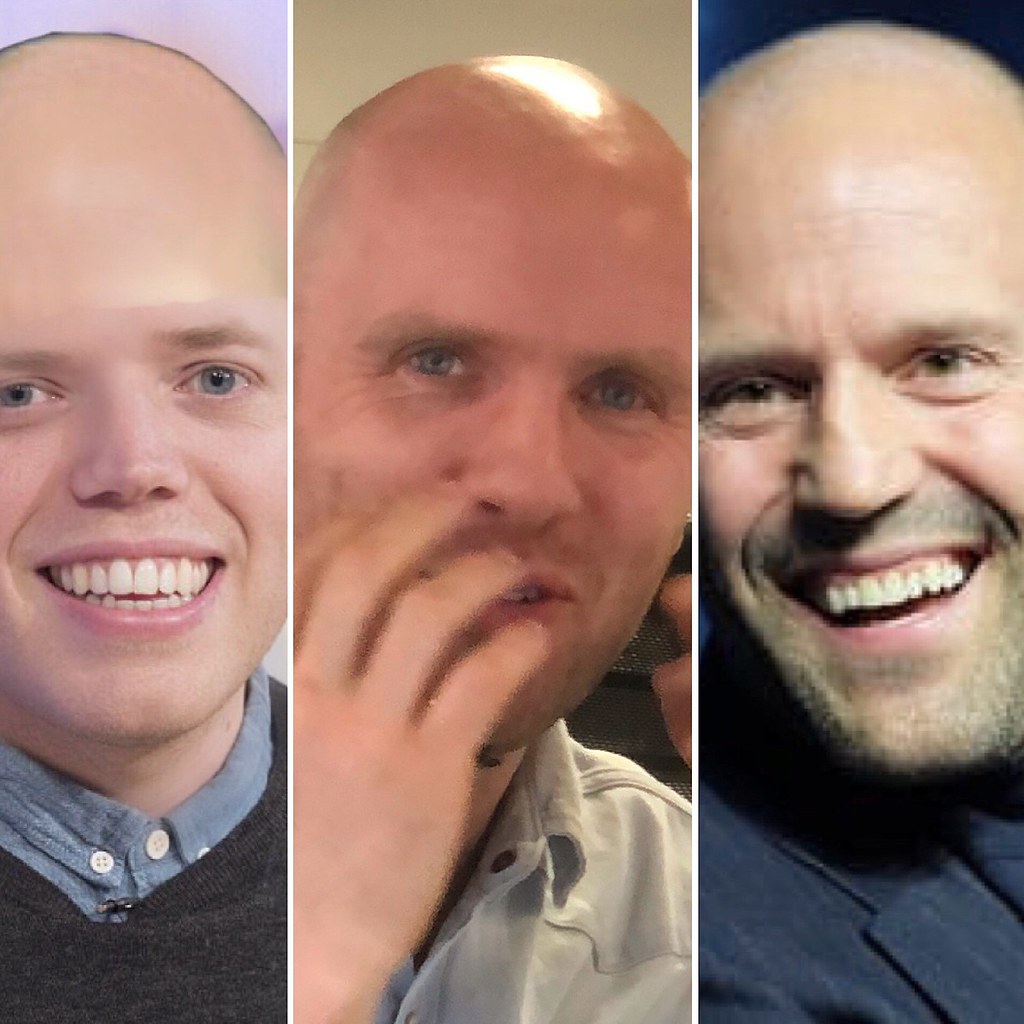The image is a vertically divided photograph featuring three close-up shots of bald Caucasian men, emphasizing only their head and upper torso. All three have distinct but similarly smiling expressions, hinting at a humorous or altered photo. The first man on the left has a big smile, blue eyes, and a notably large forehead. He wears a sweater over a blue button-up shirt. In the center, the second man, also with blue eyes and barely visible eyebrows, has a slightly larger nose and has his hand up to his face, giving a thoughtful expression. He wears a gray collared shirt. The third man on the right sports a pointy nose, small brown eyes, a huge smile, a slight stubble beard, and is dressed in a gray suit coat. His head is turned slightly to the left, capturing a joyful moment. While it's suggested that all three images might depict the same individual, subtle differences in expressions and attire might hint otherwise. There is no text within the image.